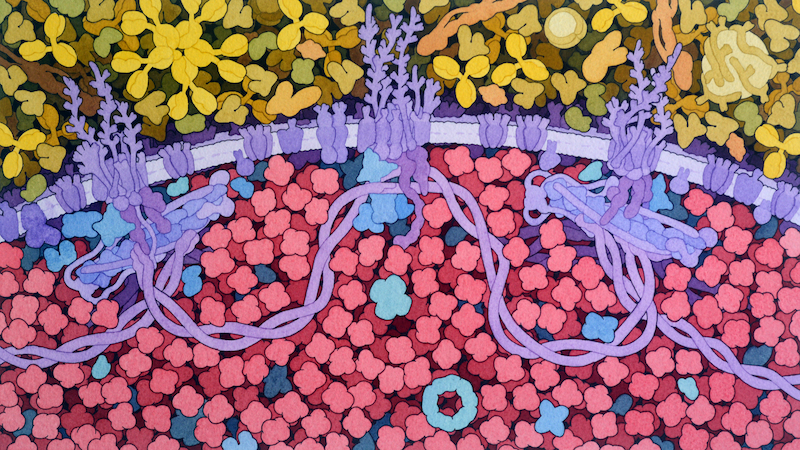The illustration features a diverse array of abstract shapes and designs. Towards the top, there are yellow and green shapes resembling leaves or pods, often grouped in clusters of three connected by stalks. Cutting across the center of the image is a purplish band that curves upward, composed of a light purple line adorned with darker purple leaves. Below this, a twisted double strand reminiscent of a loosely wrapped DNA helix or rope spirals around. 

The bottom portion is dominated by pink and red shapes, many of which resemble four-leaf clovers. Interspersed among them are a few pieces in bluish-green and light purple, with some of the purple shapes appearing underneath the others. In the bottom center stands a notable bluish circle. Abstract and richly textured, this illustration juxtaposes organic forms with intertwining strands and vibrant color contrasts.